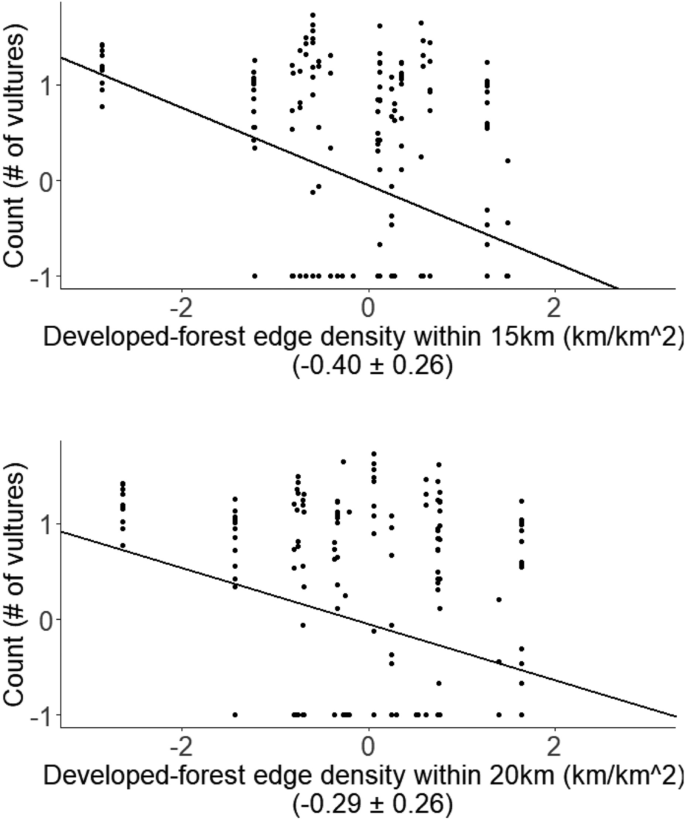The image features two stacked bar graphs commonly found in academic articles, each illustrating the relationship between vulture populations and the density of developed forest edges over two different distances. Both graphs share a vertical axis labeled "Number of Vultures," with values ranging from -1, 0, to 1, while the horizontal axes indicate "Developed Forest Edge Density," with increments from -2, 0, to 2.

The top graph measures the forest edge density within 15 kilometers. It shows a line extending from the top left (above the -1 mark) to the bottom right, past the 2 mark, suggesting a steeply declining trend. Sporadically placed black dots populate areas above and below this line, providing additional data points.

The bottom graph follows a similar structure but measures the forest edge density within 20 kilometers. Here, the line also starts from the 1 mark on the left and extends downwards to the 2 mark, creating a more obtuse angle compared to the top graph. Similar to the first graph, it features black dots scattered around the line, representing variations in the data.

Overall, the graphs together depict how vulture populations vary with differing levels of forest edge density within specified distances.